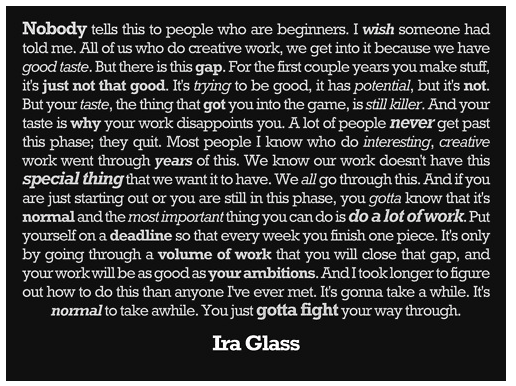**Caption:**

A minimalist black square featuring an inspirational quote in white text by Ira Glass. The message speaks directly to beginners in creative fields, emphasizing the importance of perseverance and the inevitability of a learning curve. Glass highlights the initial phase where one's creations may not meet their own high standards due to a disparity between their taste and skill level. He reassures that this is a common hurdle and encourages continued effort and productivity as the pathway to improvement. The text underscores the necessity of setting deadlines and creating a substantial body of work to eventually bridge the gap between one's current abilities and their ambitions.